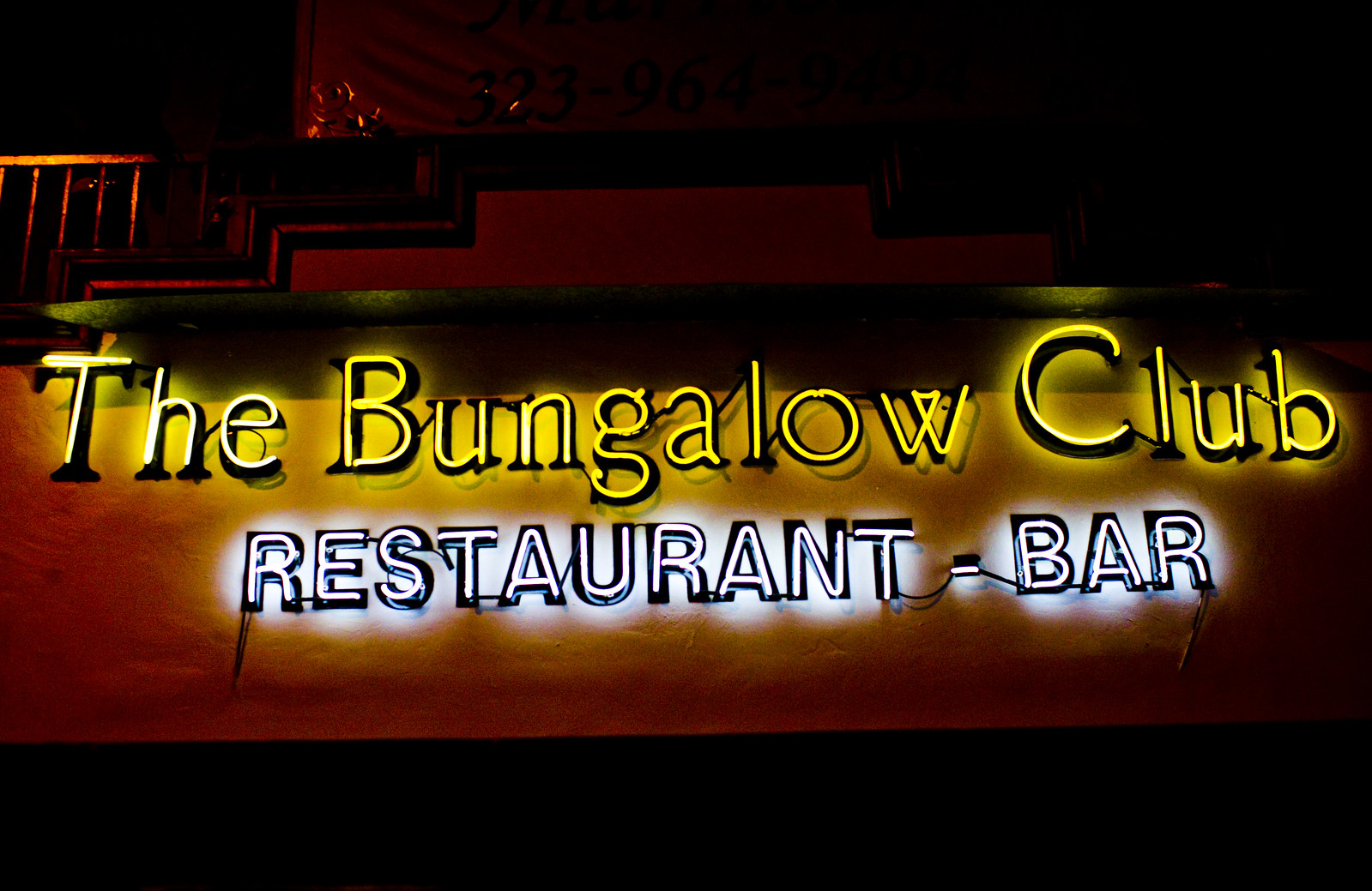The image captures a neon sign for "The Bungalow Club," taken at night, which prominently illuminates the scene. This sign, situated on the side of what appears to be a brown building with a balcony in the top left corner, features two distinct rows of text. The top row spells "The Bungalow Club" in bright yellow neon, with uppercase letters for the first letter of each word, casting a soft yellow glow on the brown rectangle backdrop. Below, "Restaurant-Bar" is written in white neon, in all-uppercase letters, emitting a soft white glow that reflects off the wood behind it. The overall atmosphere of the image hints at a dark area of town, with possible red hues from street lighting contributing to the ambiance. The neon sign, with its bright and colorful lights, stands out prominently against the dark background, creating a captivating nighttime scene.